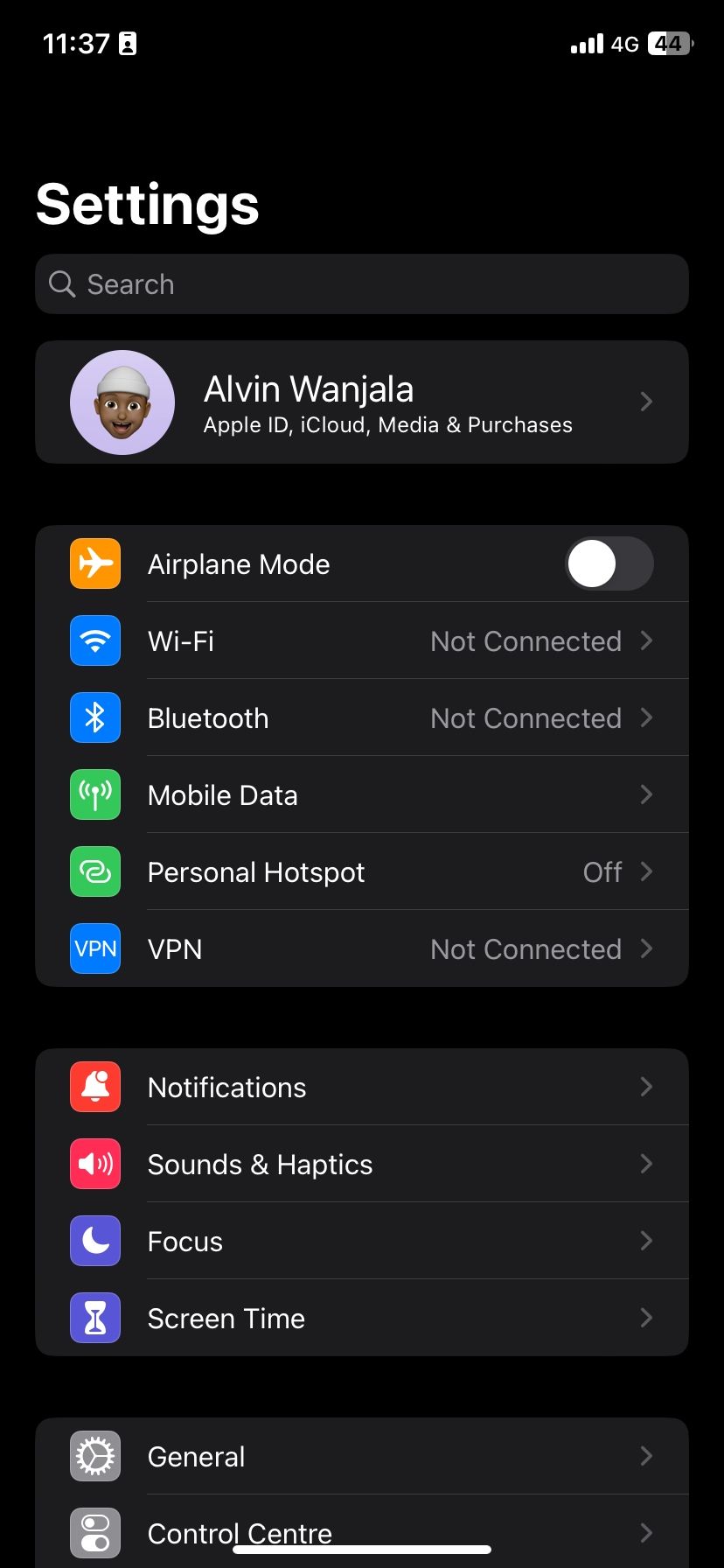A detailed screenshot taken with a smartphone showcases various elements indicative of a settings menu interface. On the left side of the screen, the time is displayed in white text, reading "11:37." The upper right corner features several indicators: a Wi-Fi icon, a "4G" label, and a half-full battery icon colored in white and gray, with "44" in black text overlaying the battery symbol.

Dominating the upper portion of the screen, the large, bolded, white title "Settings" stands prominently. Below it is a dark gray, rectangular search bar extending nearly the full width of the screen, featuring a light gray magnifying glass icon on the left and "Search" text beside it.

Further down, a circular profile picture with a lilac background displays a smiling face. Next to this profile, the user's name is written in light gray. The main portion of the screen lists various smartphone settings, each with square-shaped icons on the left and corresponding labels in the center. The settings options include: Airplane Mode, Wi-Fi, Bluetooth, Mobile Data, Personal Hotspot, VPN, Notifications, Sounds and Haptics, Focus, Screen Time, General, and Control Center. The menu is set against a black background, making the white text and icons stand out clearly.